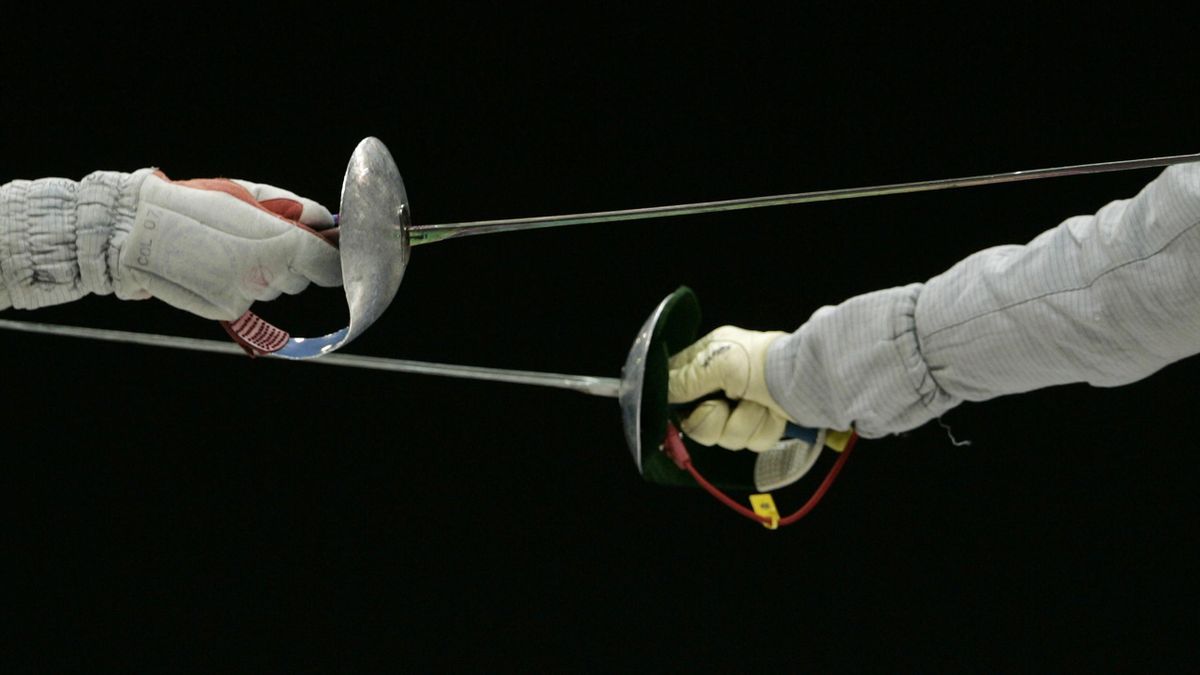This close-up photograph captures an intense moment in a fencing competition, focusing solely on the forearms and gloved hands of two fencers, poised with their silver fencing swords against a stark black background. The tension is palpable as the swords, with their handles nearly touching and protective shields just inches apart, crisscross in the center of the frame. On the left, the fencer's padded forearm extends into a gray glove marked by red highlights and a grip adorned in shades of blue and red. On the right, the competing fencer's forearm is similarly padded, leading into a white leather glove. The black-padded shield of their sword features a red cord trailing from the epi into their sleeve, hinting at the technical intricacies of the sport. Both swords are partially obscured beyond the hands, emphasizing the protective gear and readiness of the athletes at this gripping moment.